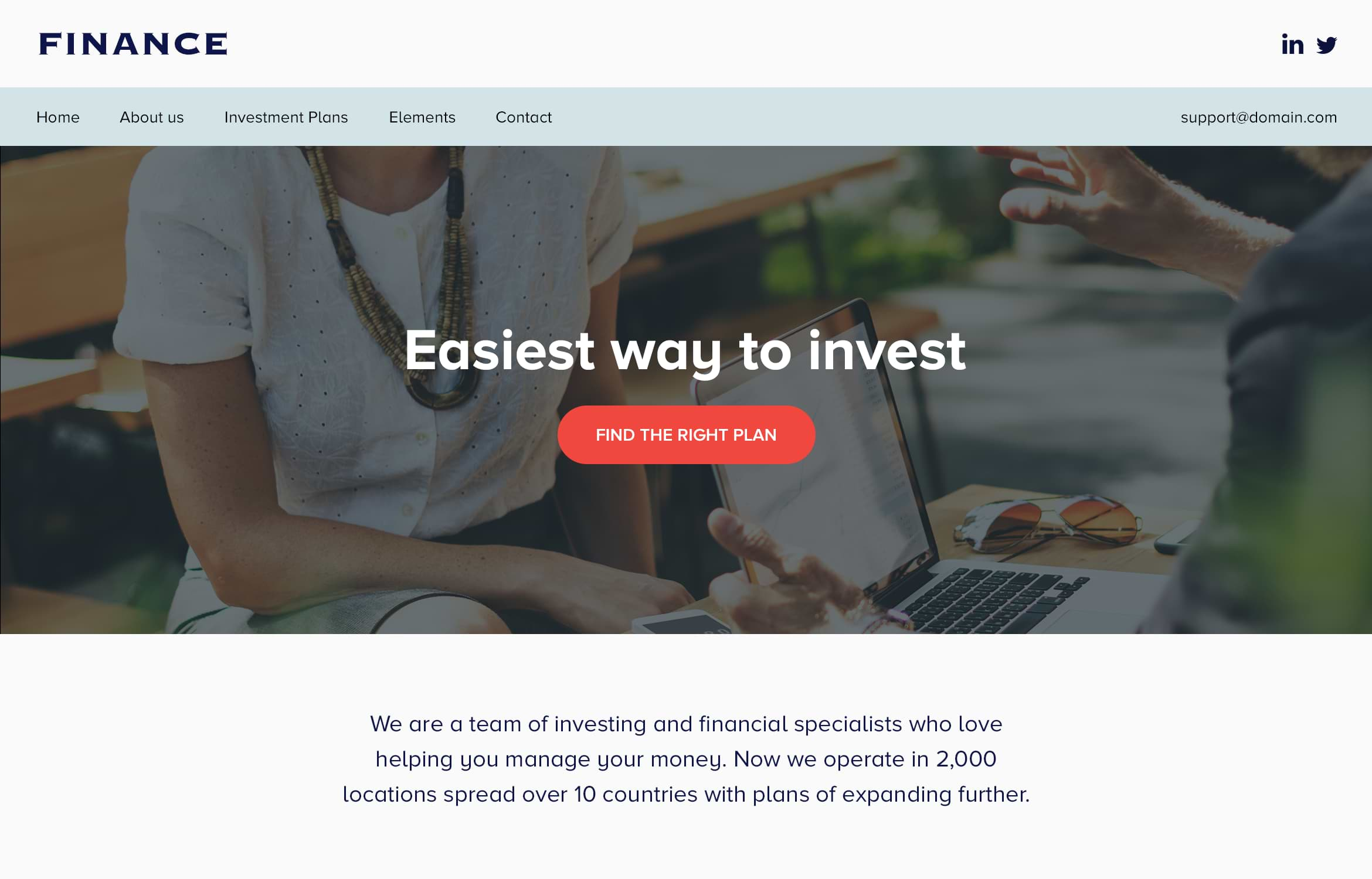In the top left corner, bold text reads "Finance." Below this, a horizontal light blue search bar features options: "Home," "About Us," "Investment Plans," "Elements," and "Contact." On the far right, "support@domain.com" is displayed. 

Below the search bar, an image depicts a man sitting at a desk with a laptop and a pair of sunglasses placed on it. The man, gesturing with one hand as if speaking, seems to be engaged in conversation with a woman across from him. The woman is dressed in a short-sleeved white shirt and a long necklace, with her hands resting on her lap. In the background, a picnic table area is visible. 

Overlaying the image, white text states, "Easiest way to invest." Below the image, in gray text, it reads: "We are a team of investing and financial specialists who love helping you manage your money. Now we operate in 2,000 locations spread over 10 countries with plans of expanding further." Additionally, inside a long red circle, the words "FIND THE RIGHT PLAN" are written in capital letters.